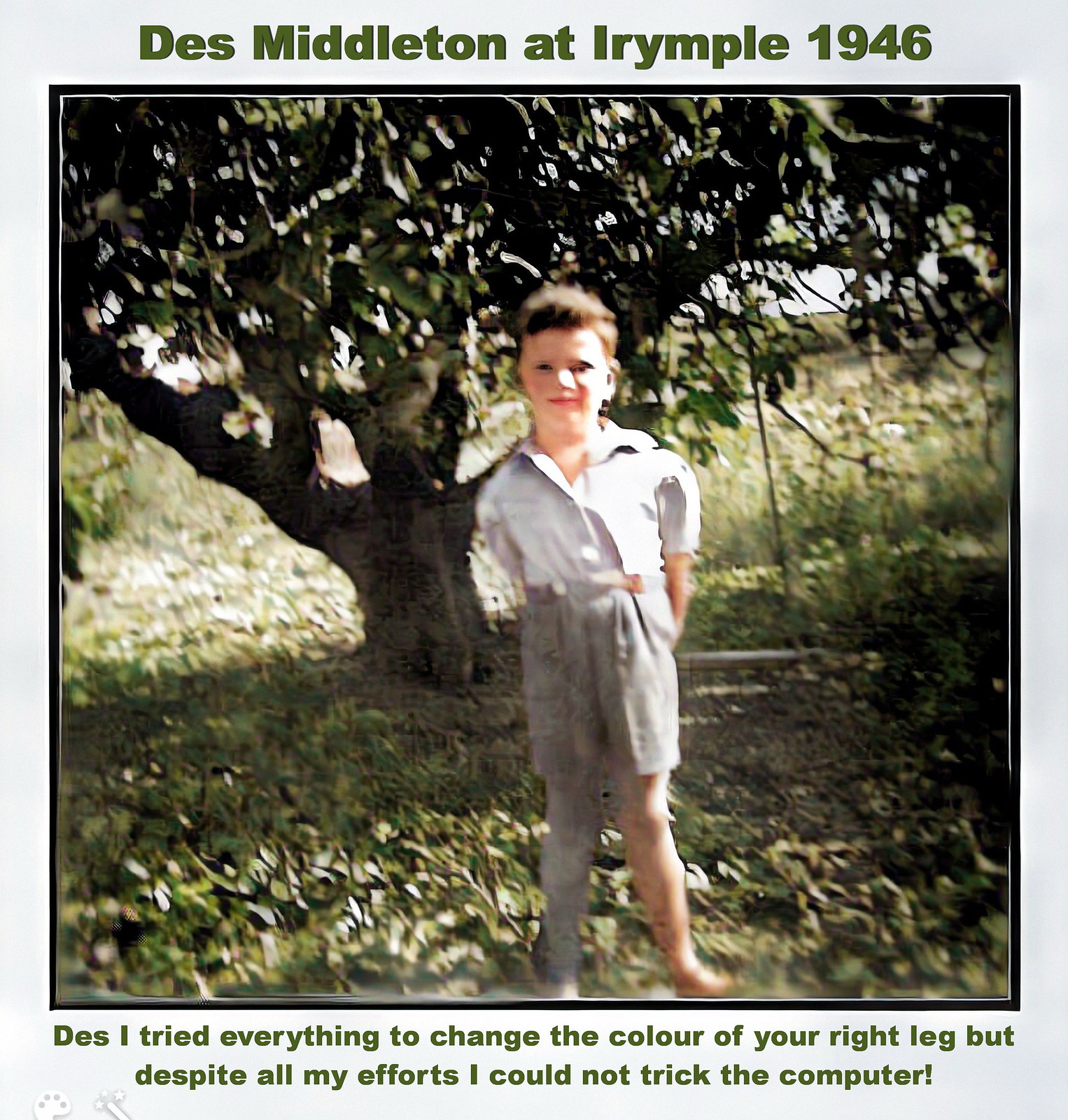The photograph depicts a somewhat blurry image of a young boy, approximately six or seven years old, standing in front of a tree with low branches. The boy, identified as Des Middleton, is dressed in gray shorts and a lighter gray shirt, with both hands positioned behind his back. He has short hair and is giving a slight smile. The image is captioned in deep green at the top with "Des Middleton at Errampul, 1946." At the bottom, it reads, "Des, I tried everything to change the color of your right leg, but despite all my efforts, I could not trick the computer," indicating that his right leg appears gray, possibly due to degradation of the color film. The photo was taken during the daytime, and Des is standing on grass with the sunlight casting a shadow to the left, suggesting it might be late in the evening.